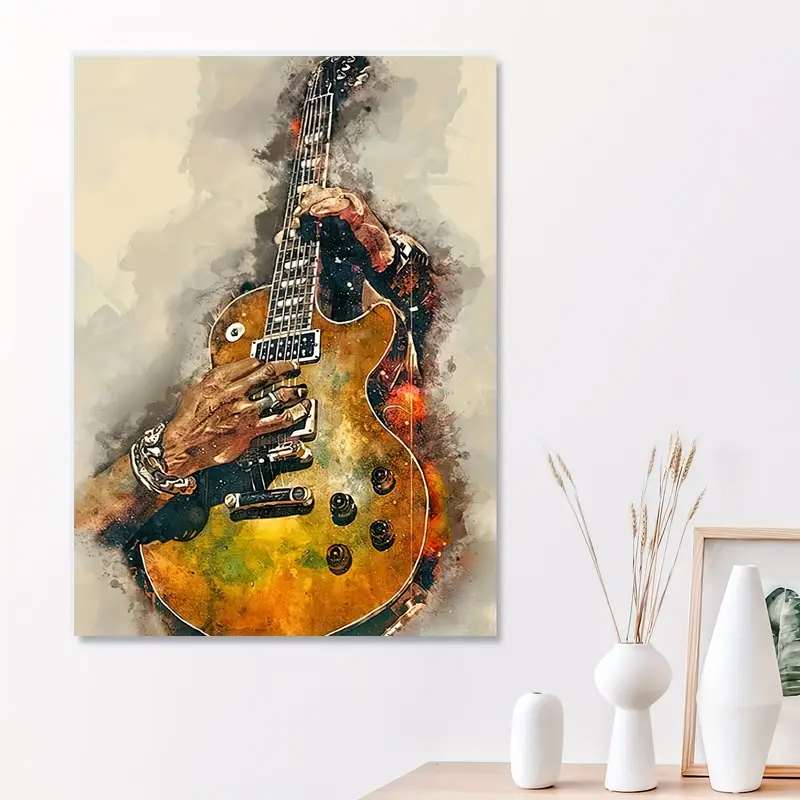The image captures a detailed painting of a famous scene depicting guitarist Slash from Guns N' Roses passionately shredding on an orange-yellowish Gibson electric guitar. In this artwork, the focus is on two hands, one at the top of the guitar adjusting the strings and the other at the bottom strumming. Notably, the hand at the top, appearing white, lacks visible clothing up to the elbow, while the black hand at the bottom is adorned with a recognizable bracelet and ring associated with Slash. The painting is set against a gray, shadowy background, enhancing the dramatism of the scene. The artwork hangs frameless on a white wall adjacent to a wooden table. On this table, there are several items including distinctive white vases, with the central vase having a spherical top filled with light beige wheat stalks, subtly complementing the colors of the guitar and adding to the aesthetic appeal of the setting.